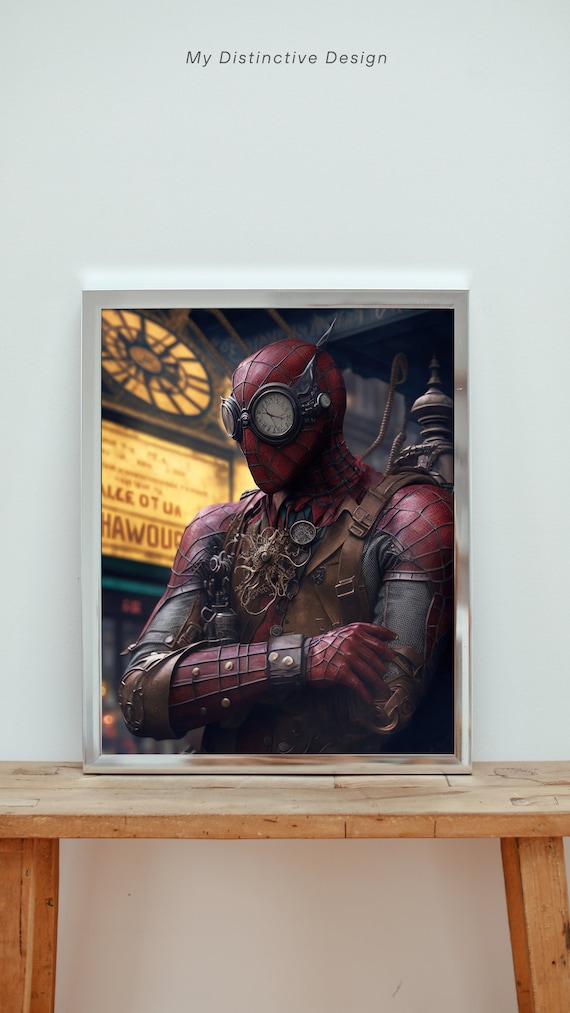In this full-color, vertically rectangular indoor photograph, the focal point is a steampunk-inspired version of Spider-Man, depicted in a toroso-up portrait. The image is prominently set against a light gray wall with thin black text reading "My Distinctive Design" at the top center. At the bottom of the scene, an unpainted, raw wooden table supports a framed picture leaning against the wall. The frame is metallic and silver, contrasting with the rich textures of the poster.

The character in the image is an alternate Spider-Man adorned in a dark, leathery red costume patterned with raised black spider webs throughout his outfit, emulating the typical Spider-Man look. However, the steampunk elements are evident: his eyes appear as clock faces rather than the usual goggles, adding an intriguing twist. Additionally, he wears a brown leather vest equipped with various mechanical accents and shoulder straps, suggesting a blend of Victorian-era aesthetics with futuristic design. His arms are folded, and the ensemble includes a pendant or piece of jewelry in the center of the vest, enhancing the detailed craftsmanship. The overall theme is dark and gritty, highlighted with yellow tones and metallic textures, which lend an industrial feel to the steampunk Spider-Man portrayal.